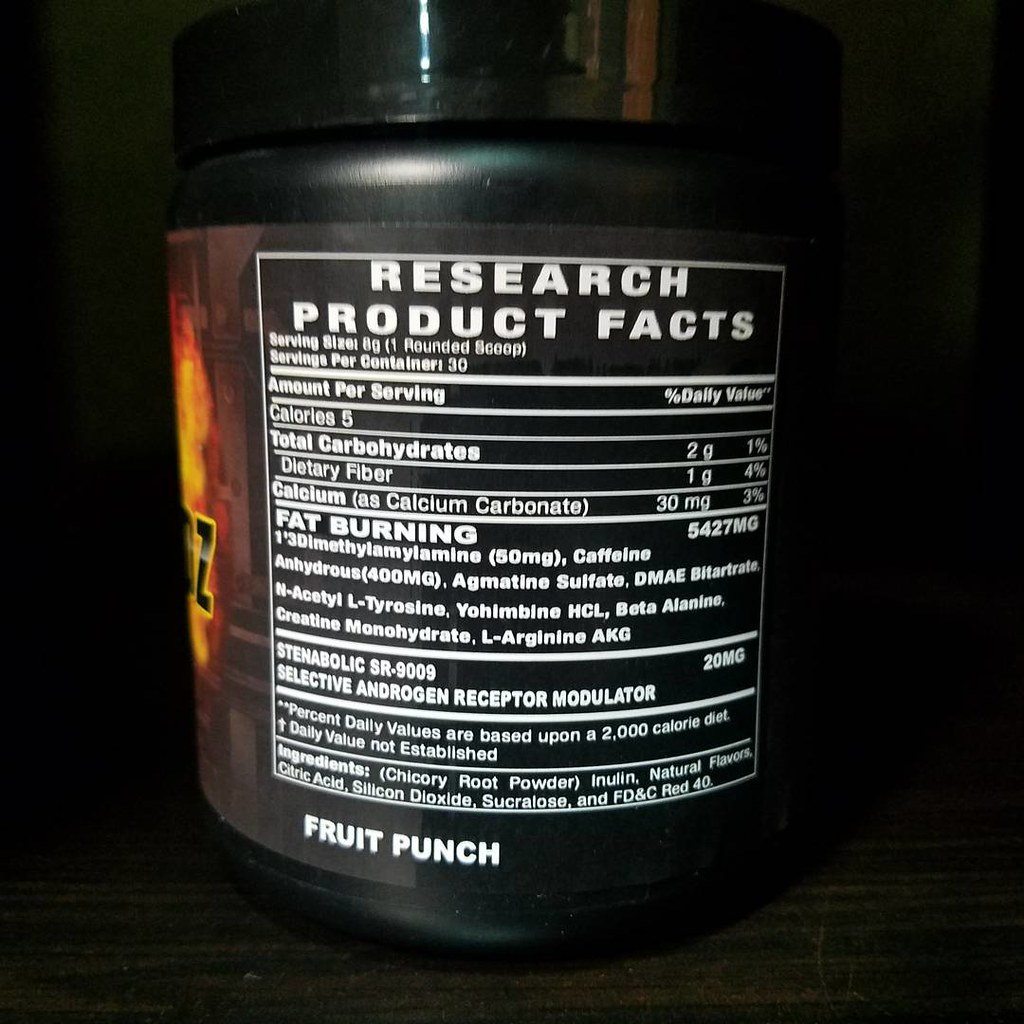This photograph features the back of a large, circular black canister filled with a powdered supplement, emphasizing its Research Product Facts. The container has a black lid and sits on a black wood surface against a black background, creating a monochromatic scene. On the front of the jar, partially visible, is an orangish-red flame design, along with some steps and a hint of the letter "Z". The label details the nutrition information in white font within a white box on the black label. It states the serving size is 8 grams (one scoop), with 30 servings per container. Each serving contains 5 calories, 2 grams of total carbohydrates, 1 gram of dietary fiber, and 30 milligrams of calcium as calcium carbonate. A prominent section on the back advertises its fat-burning properties, with various ingredients listed to promote this effect. At the bottom of the label, the flavor is indicated as "Fruit Punch."